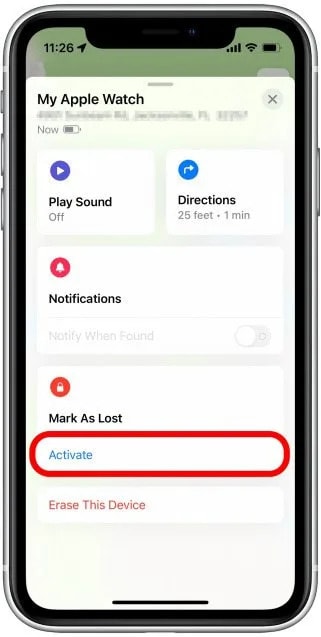The vertical image captures a smartphone encased in a clear plastic protector with black edges. The smartphone display shows various details such as the time (11:26) in the top left corner, along with a location icon. Moving to the right in the upper corner, the screen displays the signal bar icon, WiFi icon, and battery life indicator.

The content on the screen centers around an Apple Watch interface. The display features a bold heading "My Apple Watch" with a small "X" next to it, and just below it, a blurred-out section, likely an address. The battery life of the device is also shown, along with a clickable play sound icon that is currently inactive. 

The interface indicates directions with a notification stating "25 feet, 1 minute." Further down, there's a white box with a red circle containing a bell icon, marked "Notifications" in bold. The "Notify When Found" option is visible but not toggled on.

Another white box below contains a red circle with a padlock icon, labeled "Mark as Lost" in bold. The "Activate" option is highlighted in blue, enclosed in a rounded rectangular red box. Additionally, there's an option to "Erase This Device," presented in red text.

Every element of the interface is presented with clarity, making it easy to navigate and understand the various functions and statuses displayed on the smartphone screen.